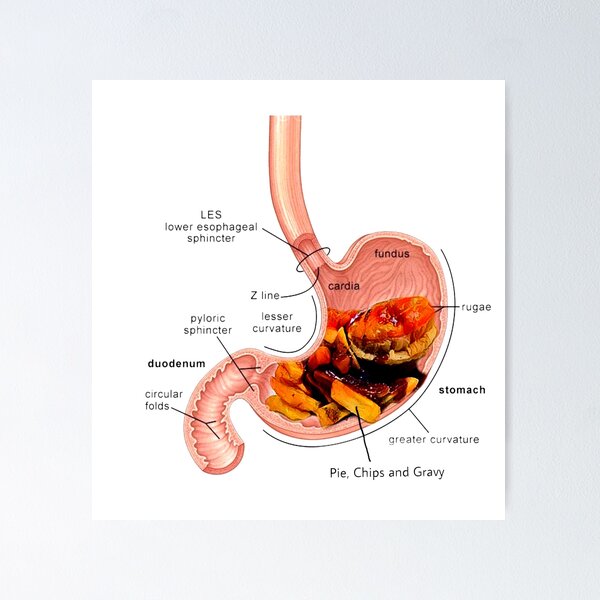This is an informational poster depicting a side view of the human esophagus, stomach, and sphincters, drawn in pink against a white background with a gray border. The diagram is meticulously labeled with medical terminology, featuring the Lower Esophageal Sphincter (L.E.S) at the top left with an arrow pointing to it, as well as other critical parts such as the pyloric sphincter, duodenum, circular folds, greater curvature, rugae, cardia, and fundus.

Inside the pink-drawn stomach, there is a colorful illustration showing a variety of undigested foods, including donuts, pie, chips, potatoes, and gravy, rendered in brown, yellow, and red to give a realistic impression of their appearance in the stomach. The labeled lines and text surround the entire diagram, providing an educational overview of both the anatomical structure and the process of digestion.